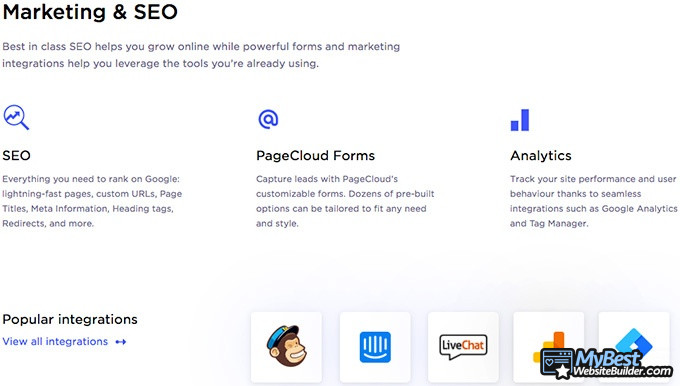The image is a screenshot of a website, featuring various blocks of black text against a crisp white background, organized into distinct sections.

At the top left corner, in bold and larger letters, the header reads "Marketing and SEO." Beneath it is a descriptive subheading: "Best in Class SEO helps you grow online while powerful forms and marketing integrations help you leverage the tools you're already using." This text is uniformly aligned to the left of the page.

Further down, the content is arranged into three vertical columns, each marked with a small blue symbol, followed by headers and brief explanations. 

1. **SEO**: The first column features a blue magnifying glass and an arrow icon pointing upward, resembling a stock ticker symbol. The title reads "SEO," and below it, the description says, "Everything you need to rank on Google, lightning-fast pages, custom URLs, page titles, meta information, heading tags, redirects, and more."

2. **Page Cloud Forms**: The second column showcases a blue ampersand (@) symbol. The header is "Page Cloud Forms," followed by the text, "Capture leads with Page Cloud's customizable forms. Dozens of pre-built options can be tailored to fit any need and style."

3. **Analytics**: The final column is marked with a blue bar graph icon, illustrating one short and one tall bar. The title "Analytics" is in bold. The accompanying text reads, "Track your site performance and user behavior thanks to seamless integrations such as Google Analytics and Tag Manager."

At the very bottom of the page, in the footer on the left side, there's the heading "Popular Integrations" in bold. Below it, a blue hyperlink labeled "View All Integrations" is presented. To its right, five icons are lined up: one of a monkey with a blue hat (likely Mailchimp), a blue speaker icon, a live chat bubble, a yellow and red bar graph, and a light blue and darker blue diamond.